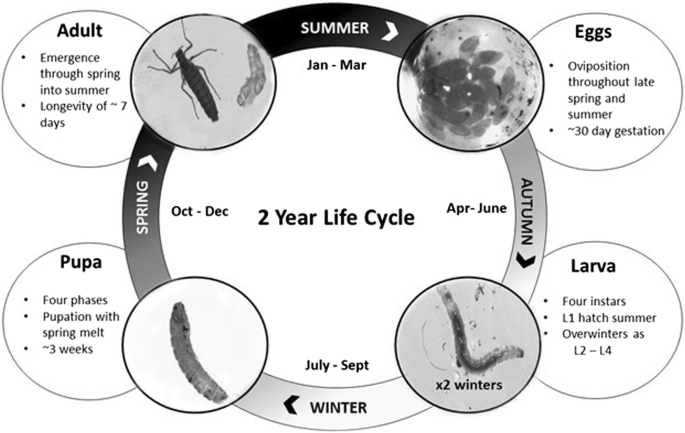The black and white infographic illustrates the detailed two-year life cycle of a beetle, visually represented in a circular format with each stage of its development marked by the seasons and corresponding months. At the center, the text "Two-Year Life Cycle" highlights the duration of this process. The cycle starts at the top with the months January through March denoting summer, moving clockwise. The right side indicates autumn with April through June, the bottom signifies winter with July through September, and the left side points out spring with October through December. 

Starting in summer, the beetle's life begins with an egg stage labeled "Eggs: oviposition throughout late spring and summer, 30-day gestation." After summer, arrows guide to autumn showing the larval stage described as "Larva: four instars, L1 hatches in summer and overwinters as L2 to L4," visually represented with an image of larval development over two winters. Following another arrow to winter, the next phase is the pupa, described as "Pupa: four phases, pupation with spring melt, three weeks." Finally, an arrow leads to spring, culminating in the adult phase labeled "Adult: emergence through spring into summer, longevity of seven days," completing the beetle's life cycle. Each stage is not only described in text but also accompanied by illustrative images, providing a comprehensive and clear depiction of the beetle's development through the seasons.